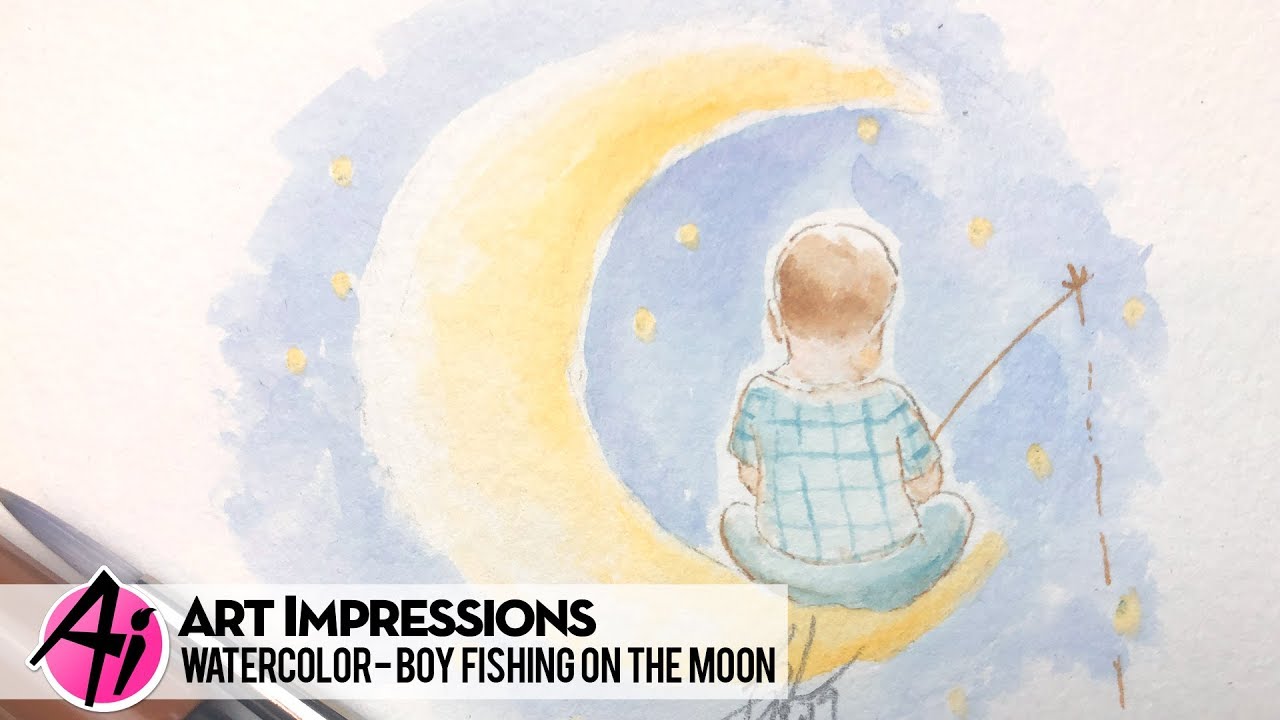This watercolor painting, displayed on a white textured piece of paper and partially visible at the bottom left corner, depicts a serene and whimsical scene. In the painting, a young boy with light blonde hair and pale skin is sitting cross-legged on the edge of a faint yellow crescent moon, which is open on the right side. The boy, seen from behind, wears a white shirt adorned with aqua-colored crosshatched stripes and light blue pants. His fishing rod extends outward, with the fishing line subtly stretching downward into the starry sky.

The sky is a gradient of light blue and purple hues, dotted with small yellow stars, creating a peaceful nighttime ambiance. To add a sense of scale and detail, the artist has signed their work just below the boy's position on the moon. The painting is bordered with a circular area of sky, beyond which the rest of the canvas remains white.

In the bottom left corner of the image, next to a pink circular logo with "AI" in black letters and a white outline, the text reads "Art Impressions, Watercolor, Boy Fishing on the Moon." A paintbrush with grayish-white bristles and a metal ring around its handle seems to rest on the canvas in this corner, adding a touch of artistic realism to the scene. This captivating artwork blends the charm of a young boy’s adventure with the tranquility of a starry night.